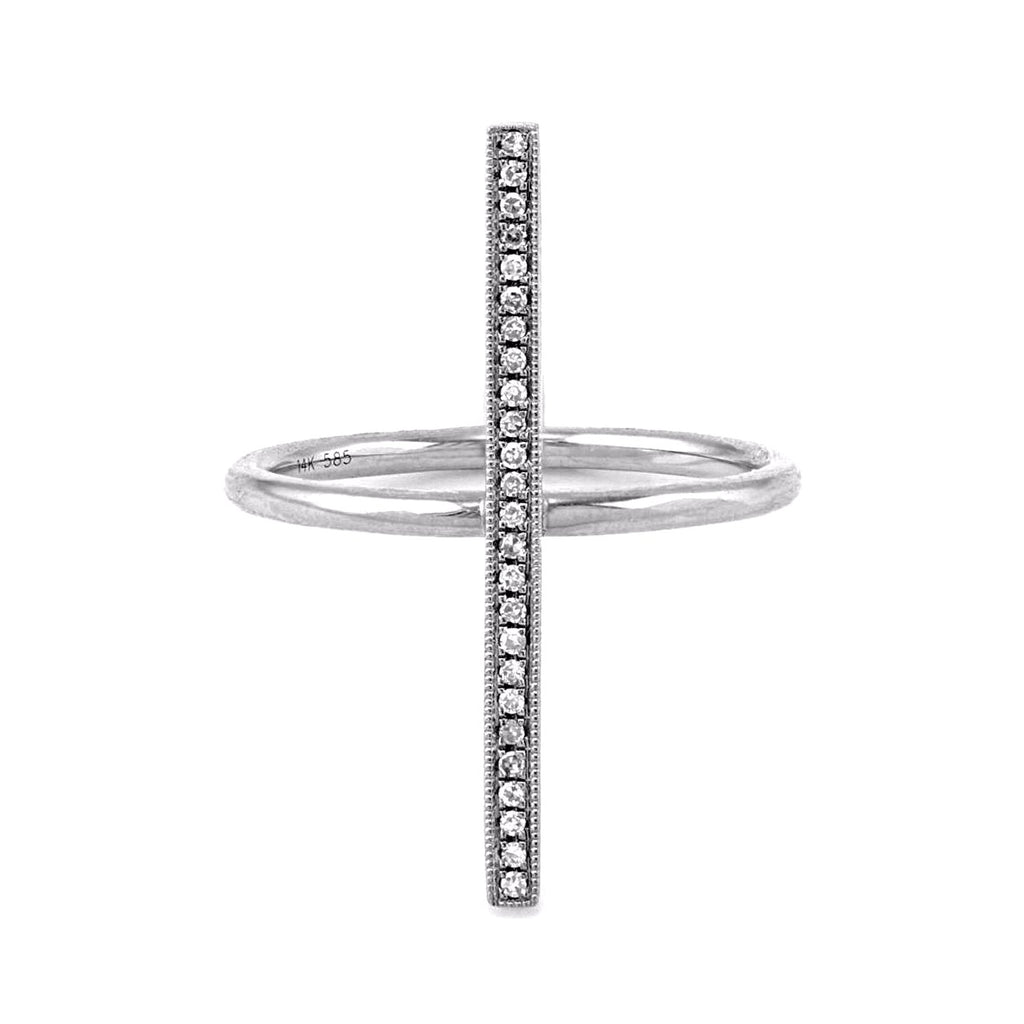This black-and-white photograph showcases two distinct pieces of jewelry. In the forefront, there is a vertically set, intricately designed diamond necklace featuring approximately 25 to 30 small, round diamonds neatly aligned. The background reveals a perfectly round ring or bracelet, likely made from a shiny, silver-like metal, engraved with "14K585" on the inside, indicating its quality. Though the black-and-white format makes it challenging to determine the exact metal, one can infer its highly polished and reflective nature. The composition is set against a white backdrop, enhancing the clarity of the diamond insets and the contrasting circular item behind the necklace.